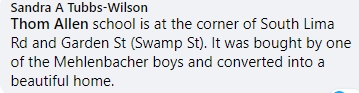This is a small rectangular image, approximately four times wider than it is tall, containing just a block of text on a very light gray background. The text is mainly in black with some parts slightly lighter. There are no additional elements or colors, only black and gray text. 

At the top of the image in a darker black font is the name "Sandra A. Tubbs-Wilson." Following this, in the next line in a darker black font, is the name "Tom Allen," which marks the beginning of a paragraph. The remainder of the paragraph is in a slightly lighter black font. It reads:

"Tom Allen School is at the corner of South Lima Road and Garden Street (Swamp Street). It was bought by one of the Mellenbacher boys and converted into a beautiful home."

This succinct block of text is the sole focus of the image, devoid of any other visual elements or variations in color.